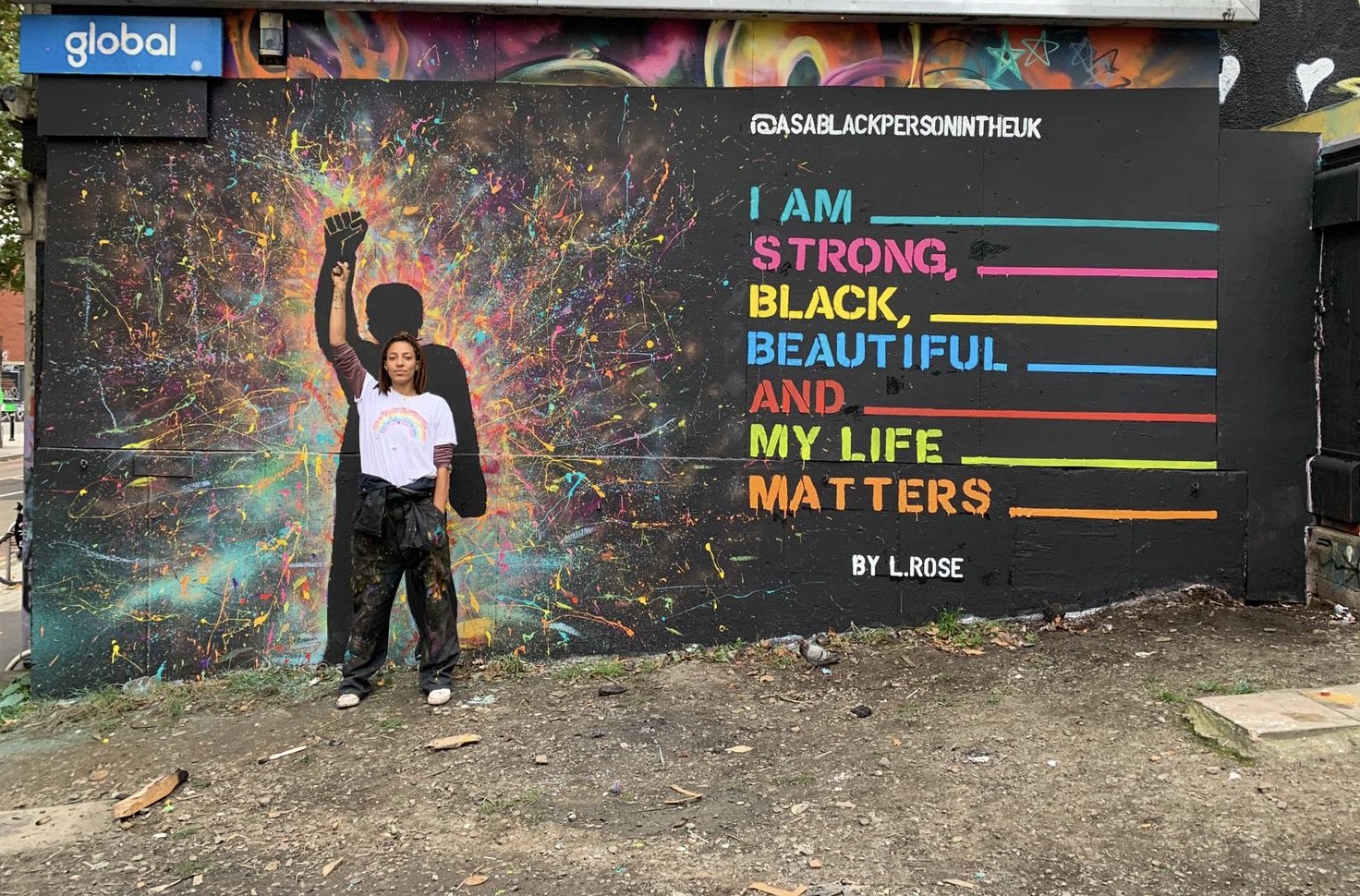This photograph captures a black woman with long, dark brown braided hair standing in front of an expressive and colorful mural. She wears a white t-shirt over a burgundy long-sleeve shirt, black paint-splattered pants, and white shoes. A jacket is tied around her waist. The mural, which she likely painted due to the paint on her clothing, features a black silhouette of a person with a raised right fist, surrounded by vibrant bursts of red, yellow, green, and orange colors against a black background. To the right of the mural, text reads, "I am strong, black, beautiful, and my life matters" by L. Rose. Additional text, somewhat obscured, appears to say "ASA black person in the UK." The setting is outdoors, in front of a building displaying the word "global" in the upper left corner. The ground beneath her is strewn with dirt, rocks, and litter, adding texture to the scene. The overall composition highlights the powerful message of the mural and the artist's pride and presence.